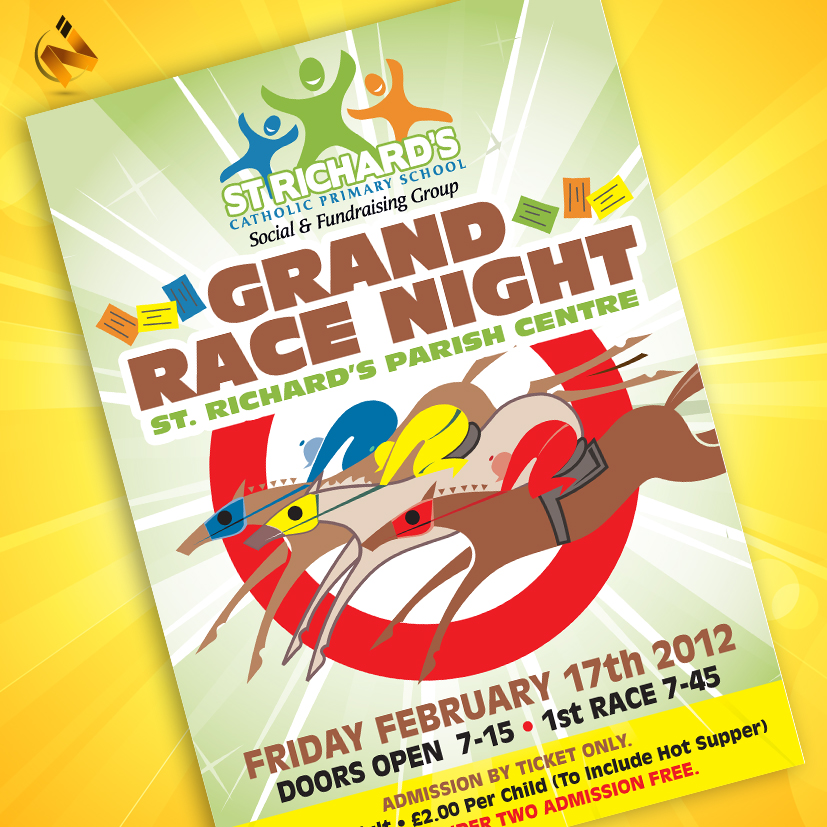The promotional poster for the Grand Race Night at St. Richard's Parish Center is framed with a yellow border and features a vibrant green background with a white sunburst at the top center. Prominently displayed at the top, it reads "St. Richard's Catholic Primary School Social and Fundraising Group." Below this, three cartoon horses, each with a rider wearing either blue, green, or orange, are depicted emerging from a red circle. The event details are meticulously laid out: "Grand Race Night, St. Richard's Parish Center. Friday, February 17, 2012." The text indicates that doors will open at 7:15 PM, with the first race starting at 7:45 PM. Admission is by ticket only, costing £2 per child, which includes a hot supper, with children under two admitted free. An additional black text further emphasizes these details. Notably, the poster includes a sideways orange "N" logo in the top left corner against the yellow background, facing towards the top left.